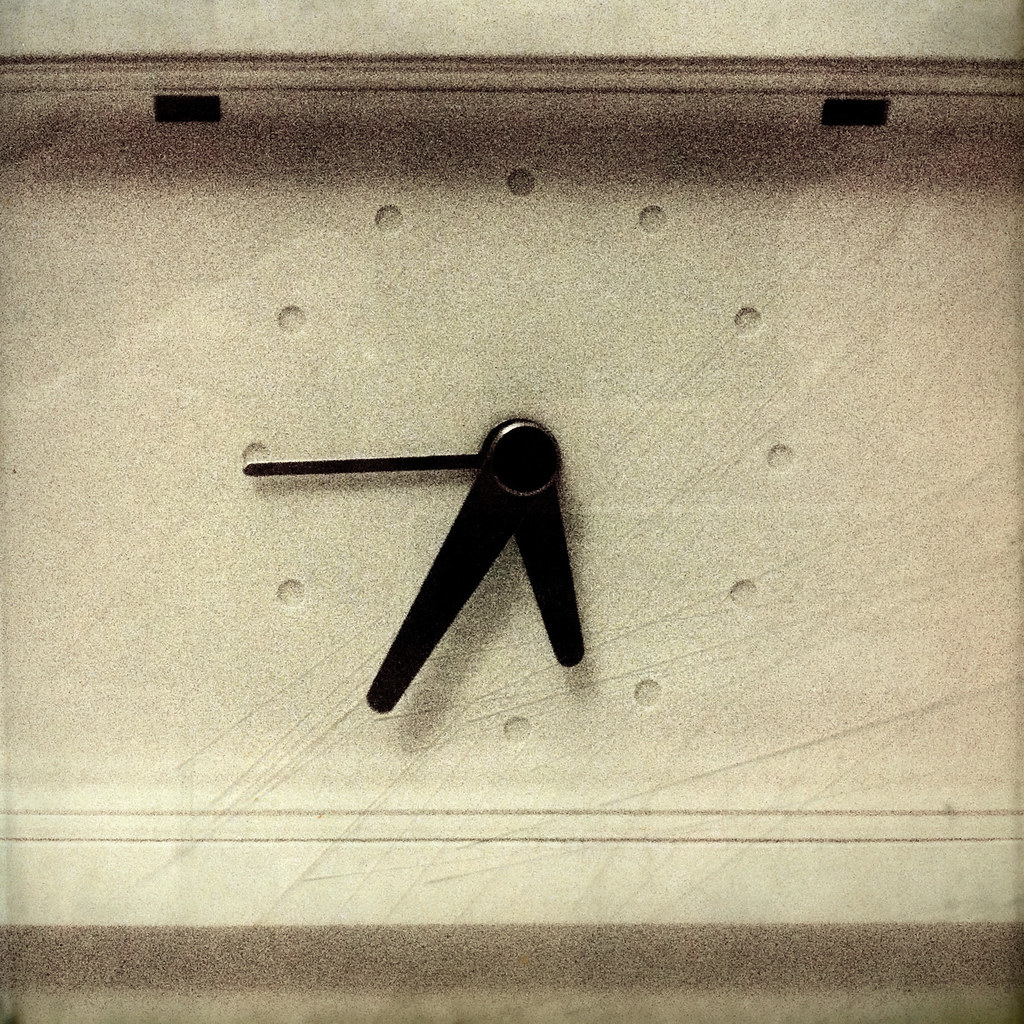This image showcases a built-in clock seamlessly integrated into a marble wall. The clock face is minimalist, featuring small, cleanly carved dots in place of traditional numbers. The clock's hour, minute, and second hands are all sleek and black, anchored by a matching black center. The marble wall, predominantly white with elegant streaks running through it, provides a sophisticated backdrop, whether or not it is actual marble. At the bottom of the clock frame, a gray bar is visible, which may be a shadow effect from the lighting or another design element.